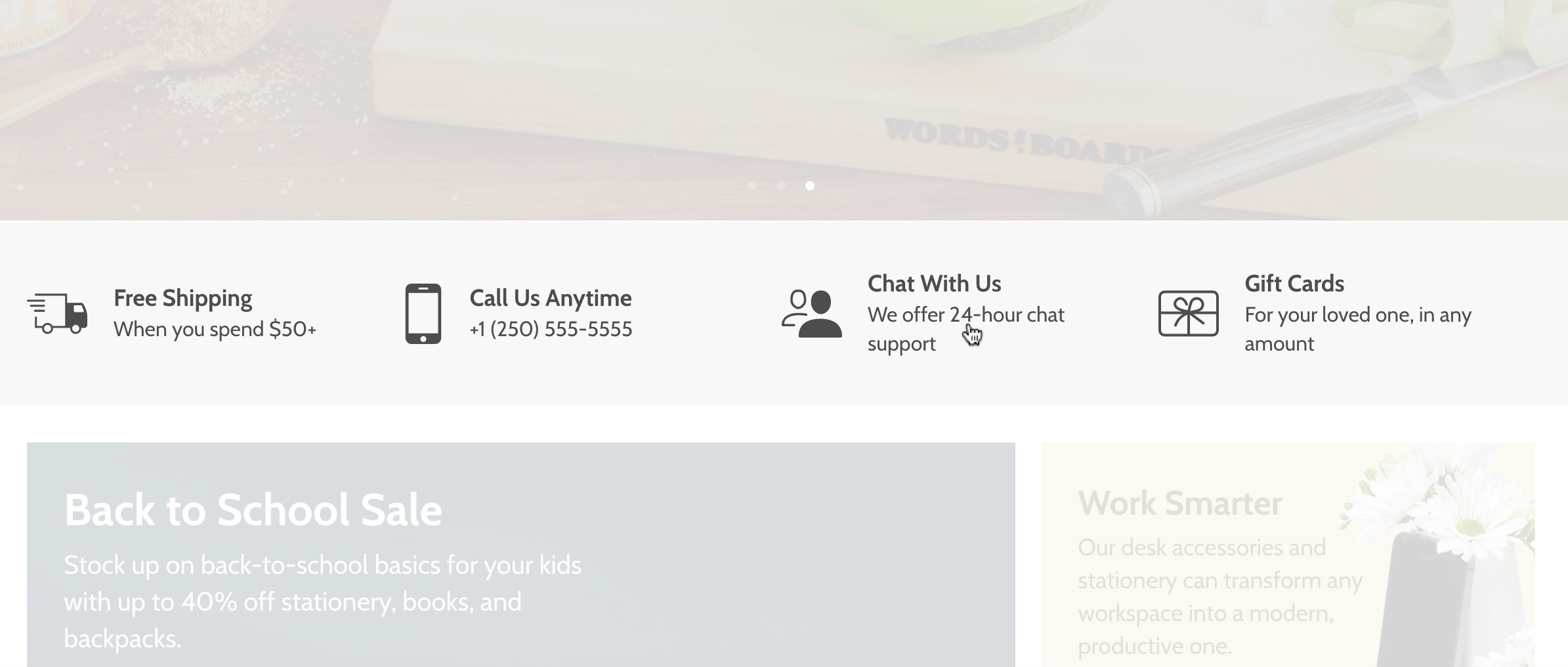The image is a collage featuring several distinct elements. At the top, there is a light purple box adorned with a delicate design consisting of variations in purple hues, darker lines, and subtle curves. In the center of this box, there's a small white circle. Some writing is present along one of the darker lines, but it is very faint and illegible. Below this, a light blue box features a small black truck with the text "Free shipping when you spend $50." Next to the truck icon is a phone symbol with the message "Call us anytime 1-250-555-5555." Adjacent to this, a chat icon with two person figures indicates "We offer 24-hour chat support."

On the right, there's a white box with a present icon and a bow, promoting "Gift cards for your loved ones in any amount." This is followed by another blue box with white text announcing a "Back-to-School Sale," encouraging viewers to stock up on school supplies, though the text is quite blurry. Finally, there is a white box containing an image of a package with flowers on top, accompanied by the text "Work smarter." Additional text is also present but is difficult to read due to blurriness.